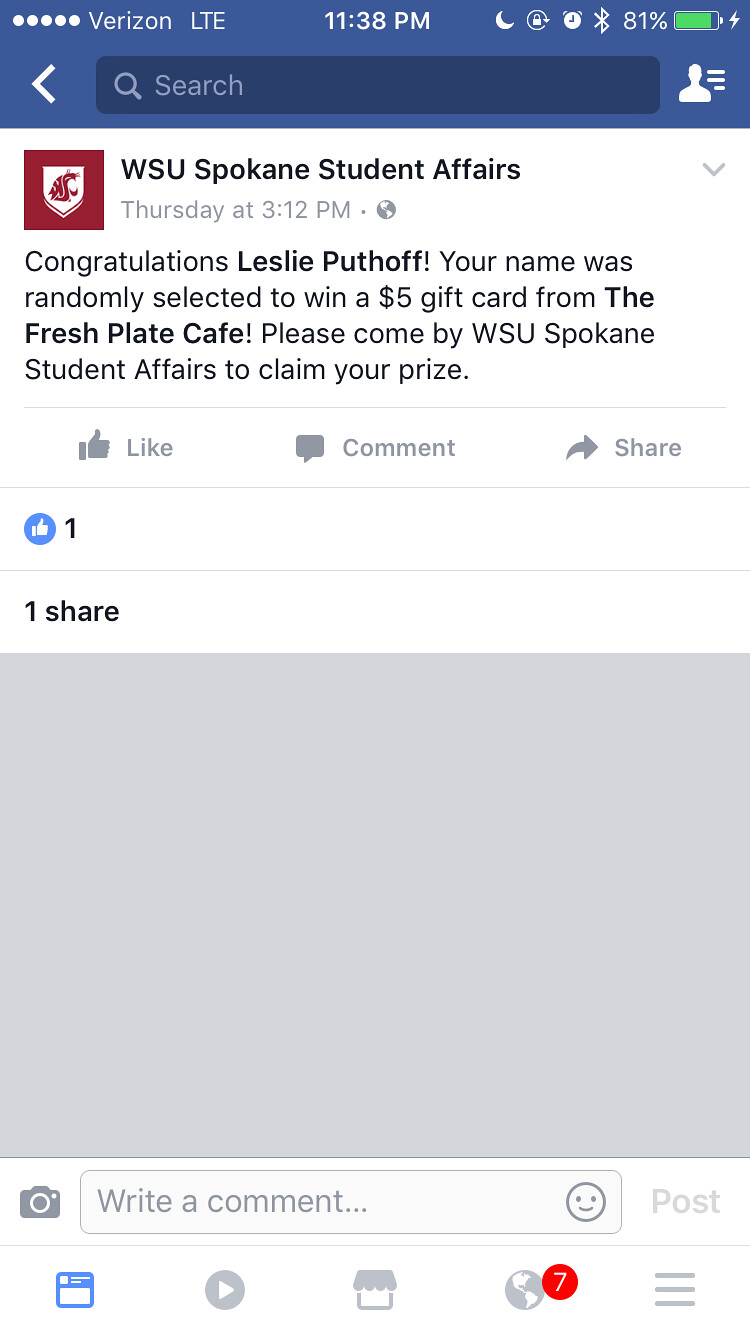The image is a detailed screenshot of a Verizon LTE cell phone, displaying a Facebook post by WSU Spokane Student Affairs. The phone shows a time of 11:38 PM, a battery life of 81%, with an active Bluetooth connection and the phone charging. At the top is a search bar with a back arrow, and directly below it reads "WSU Spokane Student Affairs" alongside the Washington State University Cougars logo in a red square. The post, dated Thursday at 3:12 PM, congratulates Leslie Puthoff for being randomly selected to win a $5 gift card from the Fresh Plate Cafe, instructing them to visit WSU Spokane Student Affairs to claim their prize. The post has garnered one like and one share. Additionally, the interface displays buttons to like, comment, and share, and at the bottom, there's a text bar for submitting a new comment. The user also has seven unread notifications indicated in the bottom right corner.